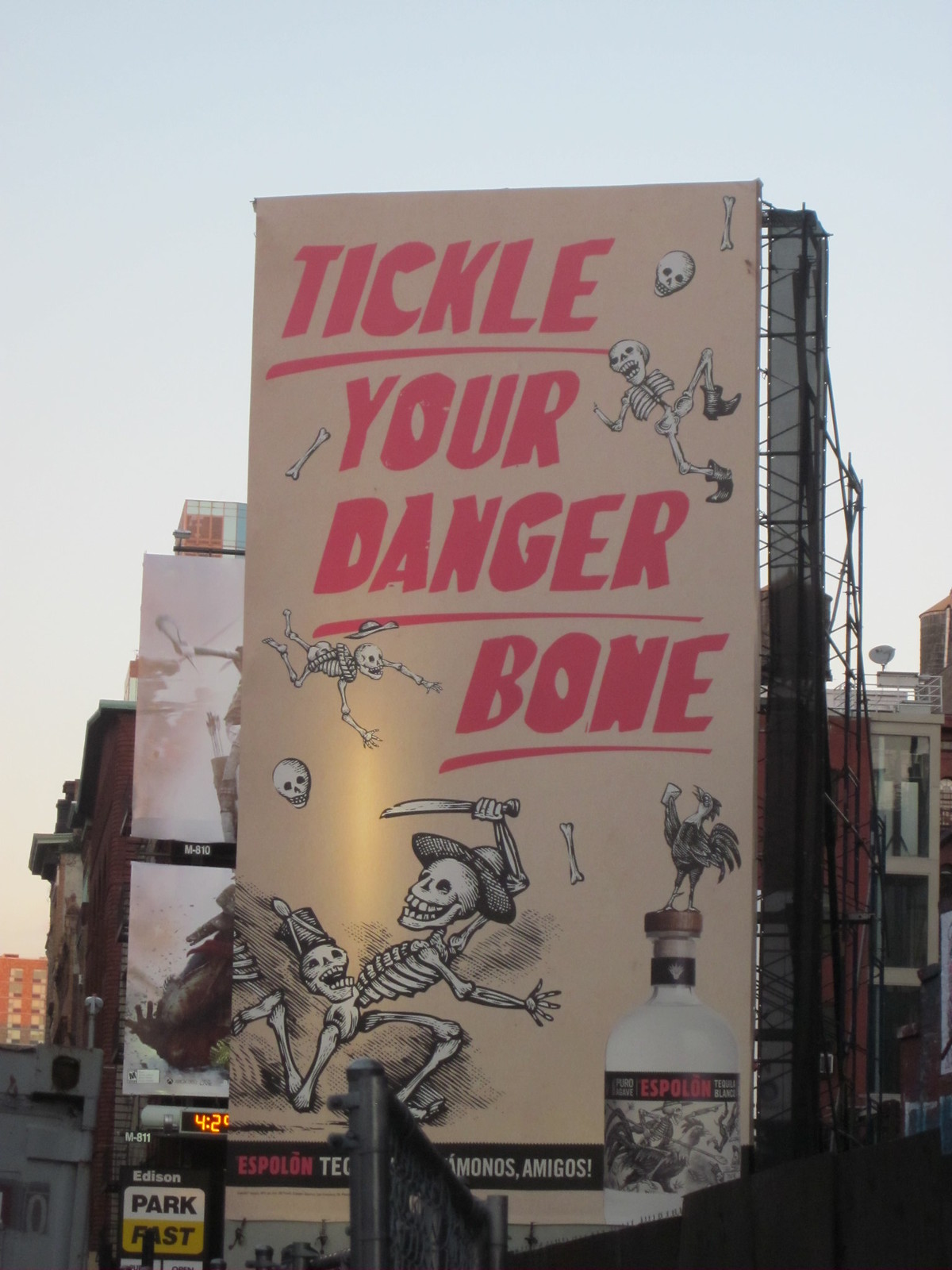The photograph captures a striking billboard perched atop a building numbered "429." The billboard, set against a backdrop of urban structures and a dusky, grayish sky, displays a vivid, somewhat macabre advertisement likely for an alcoholic beverage. The central image features animated skeletons engaged in a lively scene: one skeleton holds a knife and appears to be running towards a peculiar bottle adorned with a chicken on top. The text on the billboard reads, "Tickle Your Danger Bone. Espolón Tequila. Vámonos Amigos." Surrounding the main skeletons are additional skeletal figures clad in boots, some dancing, while another appears to be falling, donning a cowboy hat. Overall, it's an eye-catching and cool advertisement leveraging playful, thematic elements to capture attention.